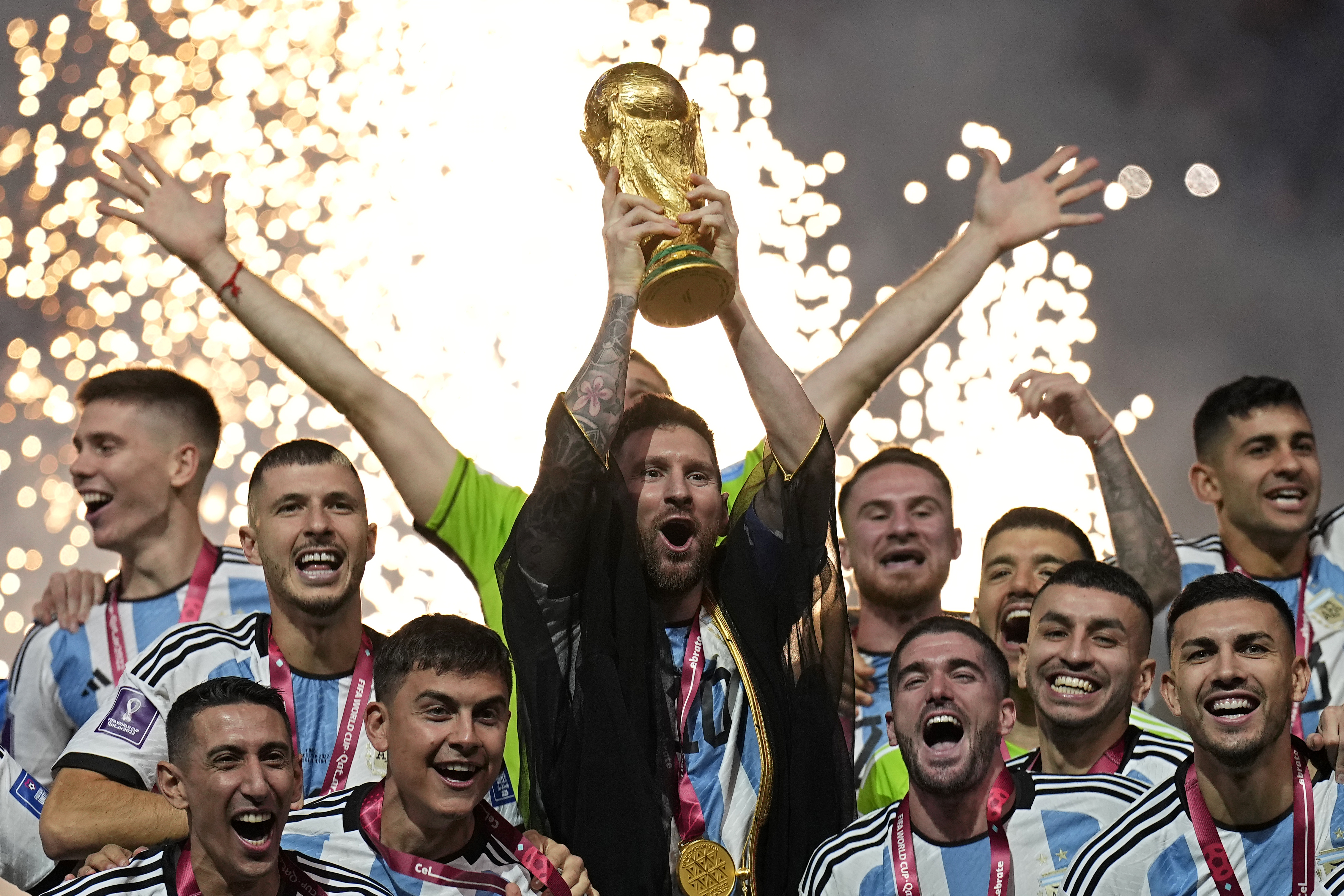In this vibrant outdoor photograph, we witness the triumphant celebration of what appears to be the Argentinian soccer team, having just won the World Cup. The image is dominated by a joyous gathering of around 12 jubilant men, all donning the iconic white jerseys with vertical light blue stripes. In their midst stands Lionel Messi, unmistakable in his transparent black robe worn over his uniform. He holds aloft the golden World Cup trophy with both hands, his face animated with euphoria, mouth wide open in a victorious roar. Around him, most of his teammates are similarly exuberant, their faces captured mid-laughter or cheer, adorned with gold medals that read "FIFA World Cup." In the background, the celebratory ambiance is enhanced by a display of bright white fireworks set against a gray sky, casting a festive glow over the scene. One man in the background stands out, wearing a green shirt and extending his arms in celebration. This photograph encapsulates a moment of sheer triumph and collective joy.